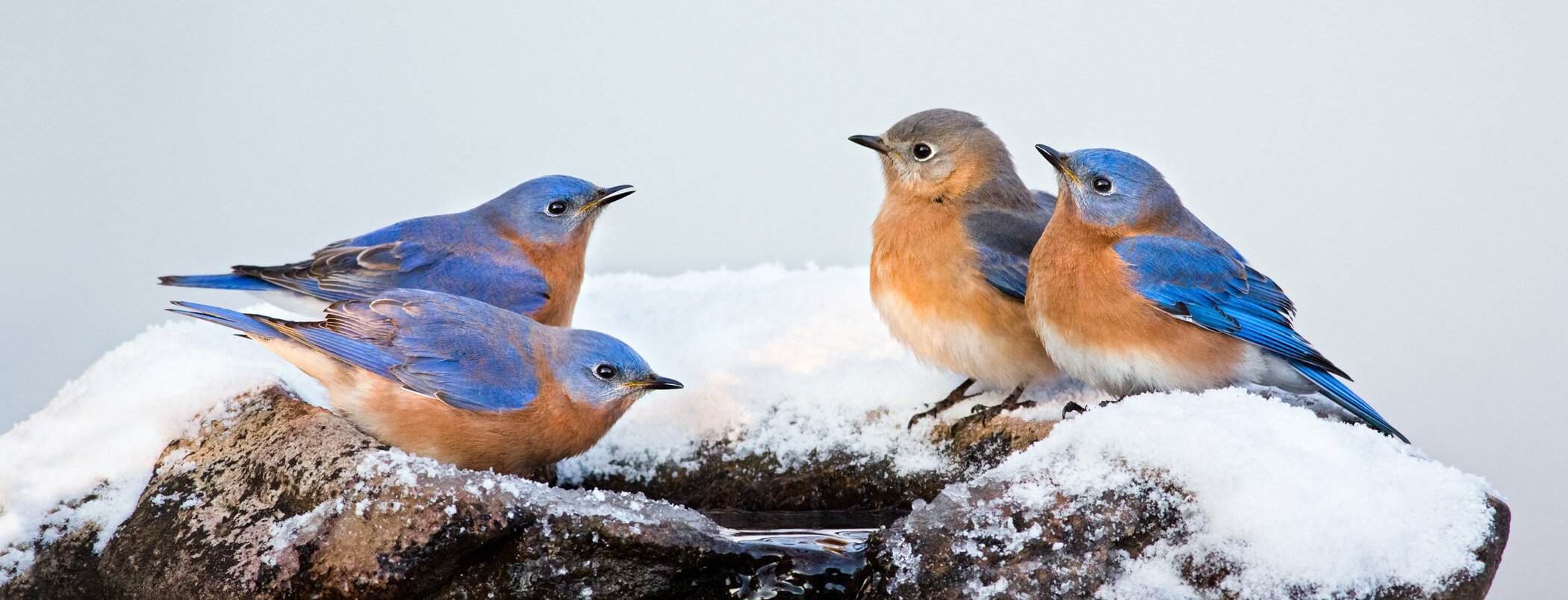The image depicts four bluebirds perched on a large, snow-covered rock or wooden stump, likely signifying winter. The rock appears to have a shallow pool of water in its center, suggesting a potential drinking spot for the birds. The background is a soft powder blue, enhancing the wintery feel.

Three of the birds feature vibrant blue feathers on their heads, orange-peach coloration on their necks, chest, and bellies, with some white mixed in. Their black beaks stand out against the snowy backdrop. On the left, one bird looks down towards the possible water source while the other gazes upwards. On the right, two other birds, with similar coloring, are both looking up and to the left, offering a view of their vibrant chest area.

The largest bird has a distinct appearance with a grayer, brownish tint to its head, making it slightly different from the others but still part of the group. All four birds appear to be of the same species, exhibiting a harmonious blend of blue, orange, and white plumage.